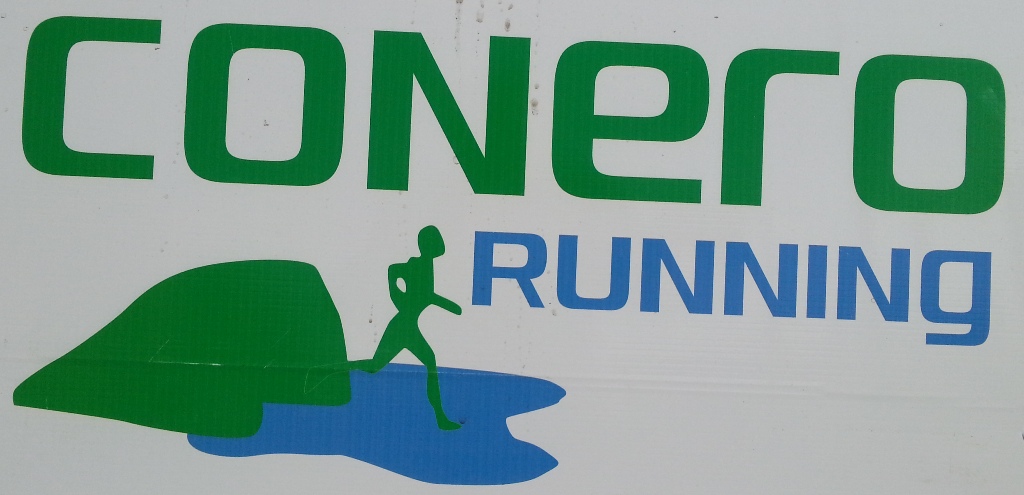The image showcases a close-up of a rectangular sign with a white background, textured with seam lines. Dominating the top half is the bold, bright green text "Conero" in all uppercase letters. Below and slightly offset to the right is the word "RUNNING" in smaller blue capital letters. To the left of the word "RUNNING" and beneath "Conero," there is a green silhouette of a running person. This figure is depicted running on a blue surface that resembles a puddle, with a green patch behind them that looks like a hill or land. The detailed design elements suggest this is likely the logo for a running company.